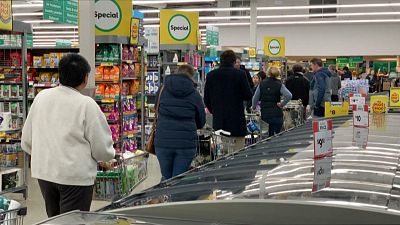This photograph captures a bustling supermarket scene, with a long line of at least six shoppers waiting to check out. Each shopper holds a basket or a cart filled with groceries. The focus is on the backs of the customers, showcasing their varied attire which suggests a cold day, with many wearing coats or long sleeves. The aisle shelves loaded with goods can be seen to the left, punctuated by bright yellow "special" signs with green borders. On the right side of the image, there are frozen food cases adorned with price tags. The supermarket is brightly lit, creating a vivid contrast between the shoppers and the stocked shelves around them. In the foreground, a person dressed in a white long sleeve shirt and black pants waits patiently, followed by a woman with a puffer jacket and a purse on her left arm, and ahead of her, a man in a black jacket, indicative of the diverse group all waiting for their turn amidst the lively supermarket environment.